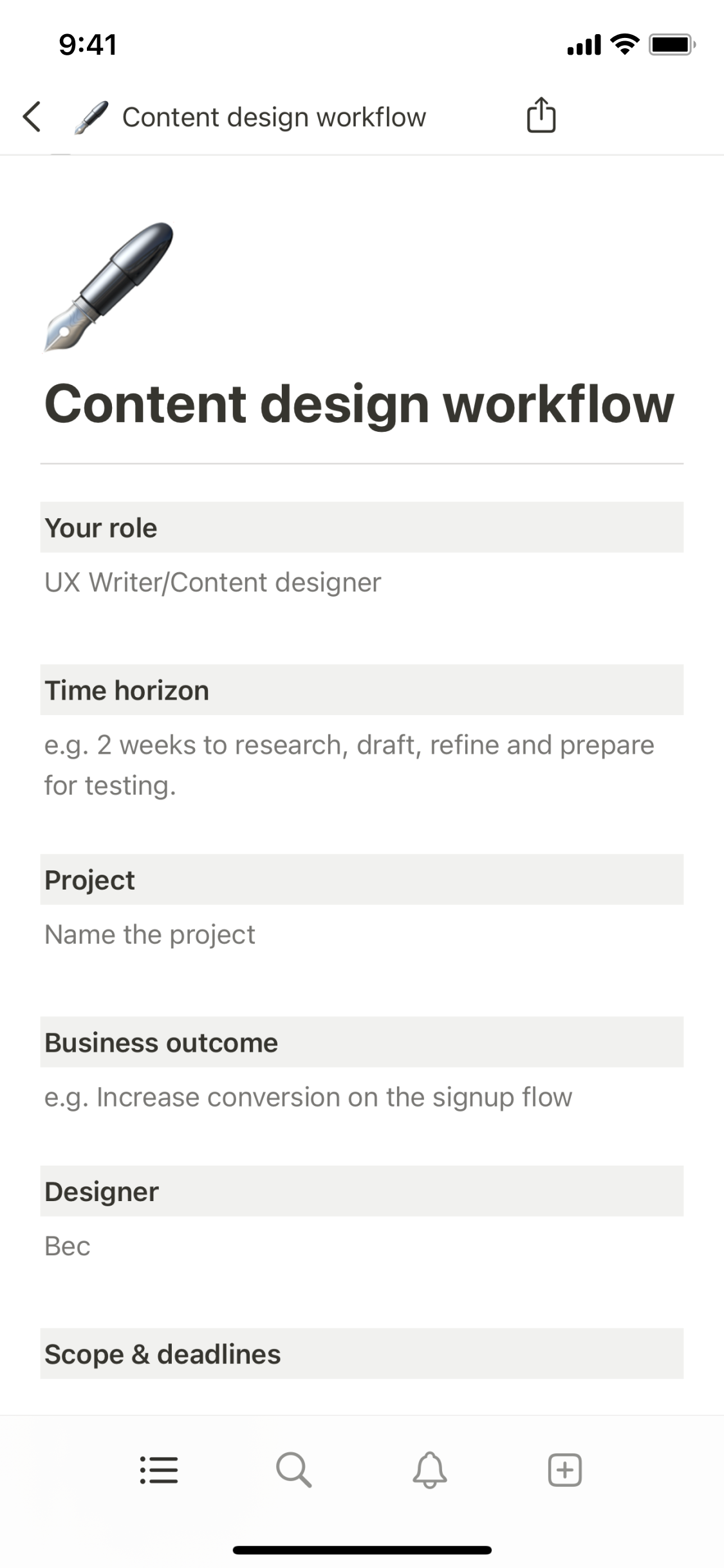This is a detailed screenshot from a cellphone displaying a content design workflow. At the top of the screen, the time reads 9:41, with indicators showing maximum cellular coverage, full Wi-Fi signal, and a fully charged battery. An icon resembling a fountain pen, tilted diagonally upward to the right, is prominently featured. Below this icon, the text reads "Content Design Workflow."

Beneath the initial header, a larger image of a fountain pen is accompanied by the heading "Content Design Workflow." The following details are listed:
- **Your role**: UX Writer / Content Designer
- **Time horizon**: For example, two weeks to research, draft, refine, and prepare for testing.
- **Project**: Name the project.
- **Business outcome**: For instance, increased conversion on the signup flow.
- **Designer**: BEC
- **Scope and deadlines**

At the bottom of the screen are icons for various functionalities:
- A bullet list icon
- A magnifying glass for search
- A bell for notifications
- A square with a plus sign in the center

This image is in a vertical orientation and contains no people, animals, plants, flowers, or trees.